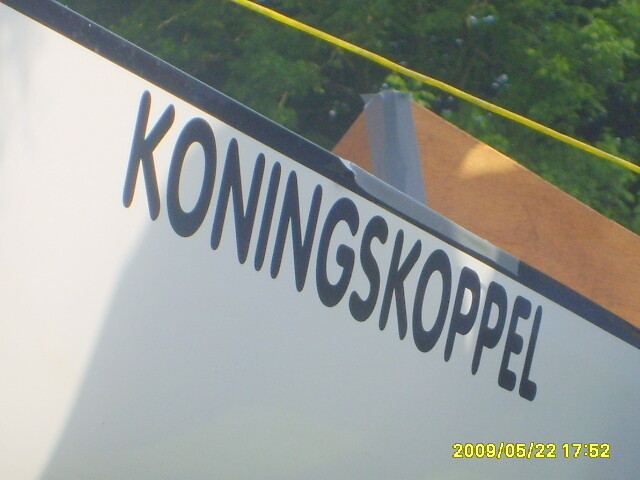The photograph captures a close-up view of a white sign, stretched diagonally from the upper left to the lower right. At the very top of the sign, there's a black trim, with the rest painted white. Black sans-serif text spells out "K-O-N-I-N-G-S-K-O-P-P-E-L," silhouetted by a shadow predominantly on the right side of the sign while light illuminates the left edge. To the upper right of the scene, a green-leaved tree is visible, suggesting an outdoor location. A yellow rope runs from the top center to the right of the image, intersecting above a smaller wooden sign below. This secondary sign appears brown and weathered, possibly secured with a piece of gray duct tape. The lower right corner of the photograph features a time stamp in small yellow text, reading "2009-05-22 1752," marking the date and time of capture. The angle of the shot and the elements in the background hint at an environment that might be close to a boat or a constructed wooden structure.